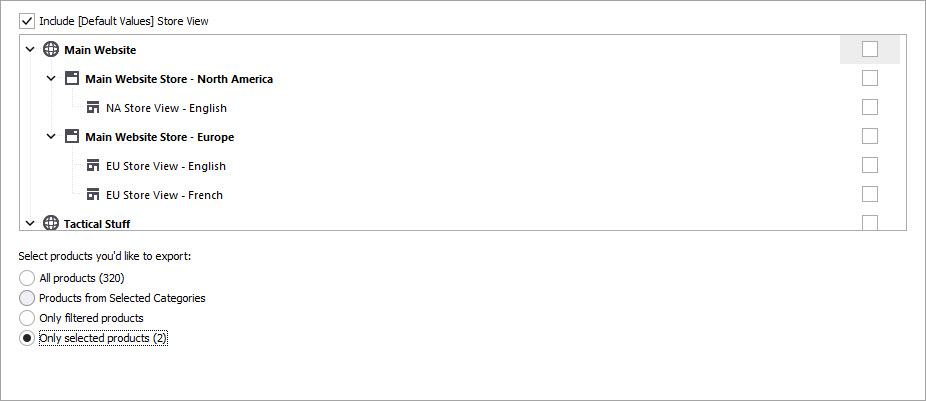In this image, the focus is on a screen displaying various settings and options for product selection. It features a white background with a thin rectangular border around it. At the top, there is a heading that reads "Include default value store view," accompanied by a check mark on the left.

Below this heading, there is a section listing different website options:
1. Main Website
2. Main Website Store North America (NA Store View - English)
3. Main Website Store Europe (EU Store View - English)
4. Main Website Store Europe (EU Store View - French)

Each option has a clickable square on its right-hand side, with only the top option highlighted in gray.

At the very bottom of this list, there is a separate category titled "Tactical Stuff."

Further down, there is a section instructing users to "Select products you'd like to export." There are four product options here, each with a circle to the left. When a circle is selected, it is marked by a black dot. The options are:
1. All products (320)
2. Products from selected categories
3. Only filtered products
4. Only selected products (currently selected with the black dot).

This detailed layout completes the image, providing a comprehensive view of the available settings and options for product selection and export.